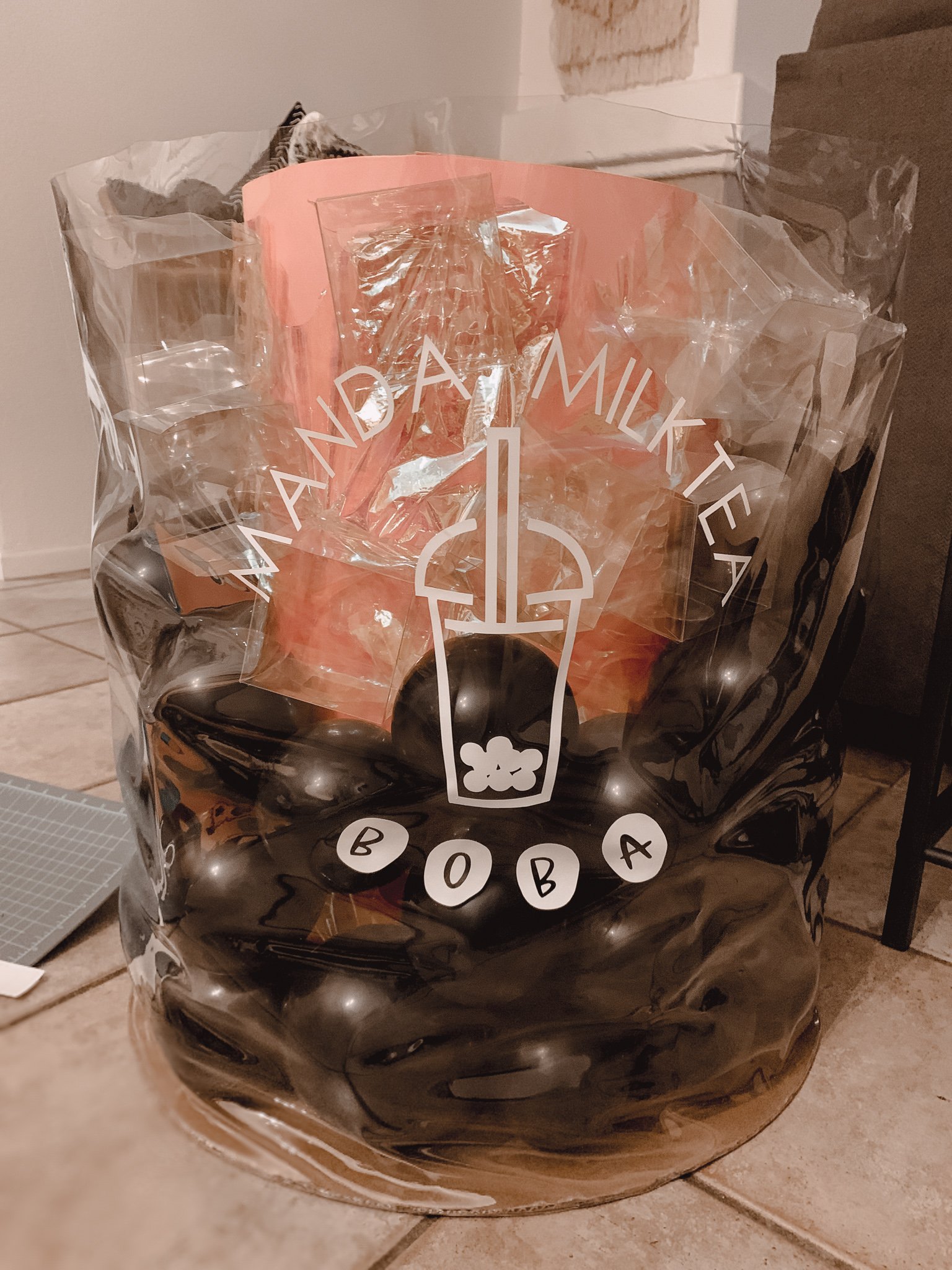This image showcases a package wrapped in clear cellophane, through which an orange piece of paper and several brown, spherical objects can be seen. The cellophane wrapping features a white font that reads "Manda Milk Tea." Additionally, there is an illustration of a glass with a straw protruding from it, containing small brown pebbles at the bottom, accompanied by the word "Boba." The package is placed on a beige-tiled surface.